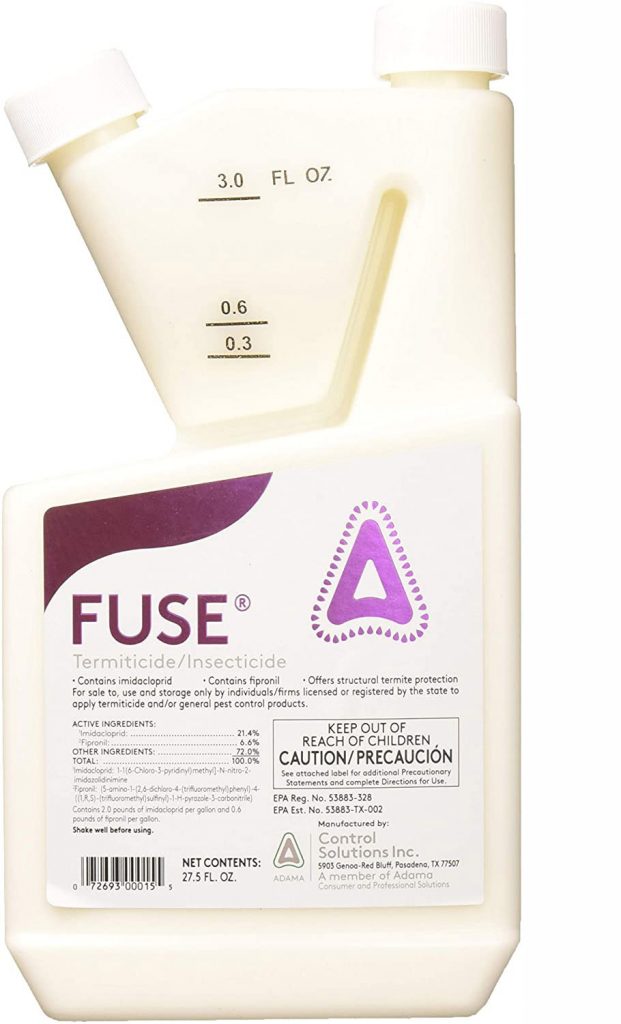This image depicts a cream-colored bottle with two white caps designed for precise measuring and dispensing. The bottle features several black markings indicating fluid ounce measurements at 3.0, 0.6, and 0.3, labeled with "FL OZ." Prominently displayed on the label, in bold purple letters, is the word "FUSE" along with a triangular logo bordered by a series of dots. Below this, the label reads "Termicide/Insecticide" in capital letters, and states it contains the active ingredients imidacloprid and fipronil. Further down, detailed information emphasizes that the product is intended for sale, use, and storage exclusively by licensed or registered individuals or firms. Additional text includes a list of active and other ingredients, amounting to a total content of 27.5 fluid ounces. The label also features a cautionary warning in a box that reads, "Keep out of reach of children," followed by "Caution Precaution." The manufacturer's name, Control Solutions Inc., is printed towards the bottom. The text is predominantly in black, contrasted by the purple elements, all on a white background, and the image also includes a barcode and some EPA regulation numbers.